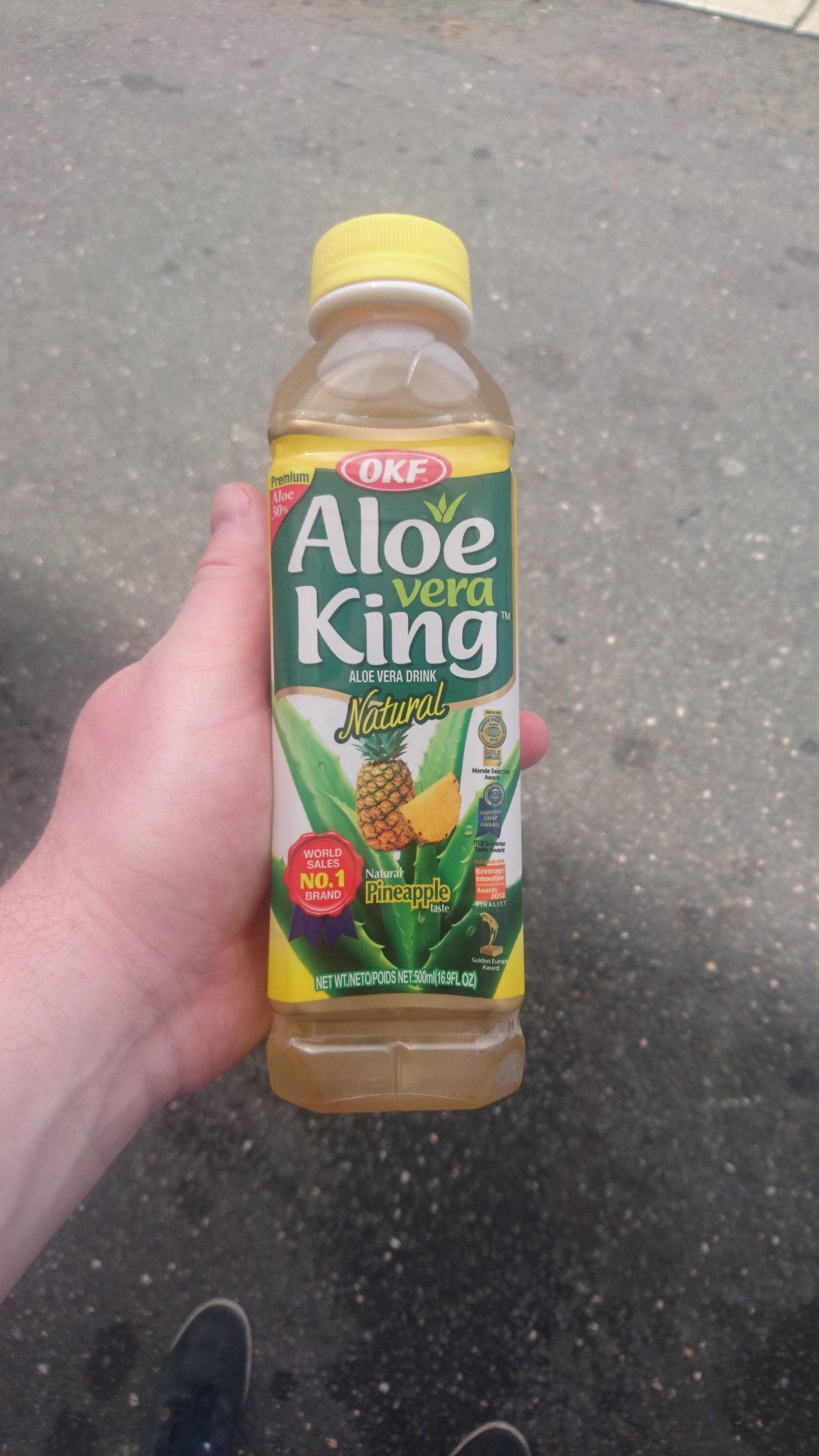In this close-up outdoor photograph, a muscular white man's hand holds a clear plastic bottle of Aloe Vera King juice. The bottle contains a gold liquid and features a yellow cap. The label is predominantly yellow and green, displaying the brand name "Aloe Vera King" and "Aloe Vera drink" in white and green letters, with "natural" in yellow beneath them. The label also includes an image of a cut pineapple nestled within a large Aloe Vera plant, along with the word "pineapple" at the bottom. A red circle indicating "number one" can be seen on the label as well. The background reveals the man's feet clad in black tennis shoes standing on worn asphalt marked with oil stains.